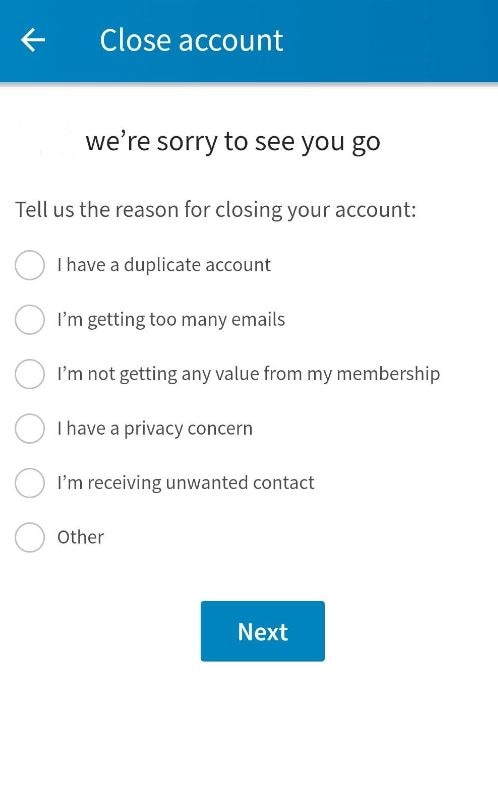The image displays an interface for closing an account. At the top, there is a prominent blue rectangular button labeled "Close Account" in white letters, accompanied by a white arrow on its left side. Below this button, in larger black font, is the message "We're sorry to see you go."

Further down, a prompt reads "Tell us the reason for closing your account:" followed by a colon. Beneath this, several reasons are listed, each preceded by a small circle for selection. The options include:
1. I have a duplicate account.
2. I'm getting too many emails.
3. I'm not getting any value from my membership.
4. I have a privacy concern.
5. I'm receiving unwanted contact.
6. Other.

These options are written in standard black font, all starting with capital letters. Finally, at the bottom of the image is a blue rectangular button with white text that says "Next." The entire interface is set against a clean white background with a very standard and frequently used font. The heading "We're sorry to see you go" utilizes a larger font size compared to the smaller text used for the details below.